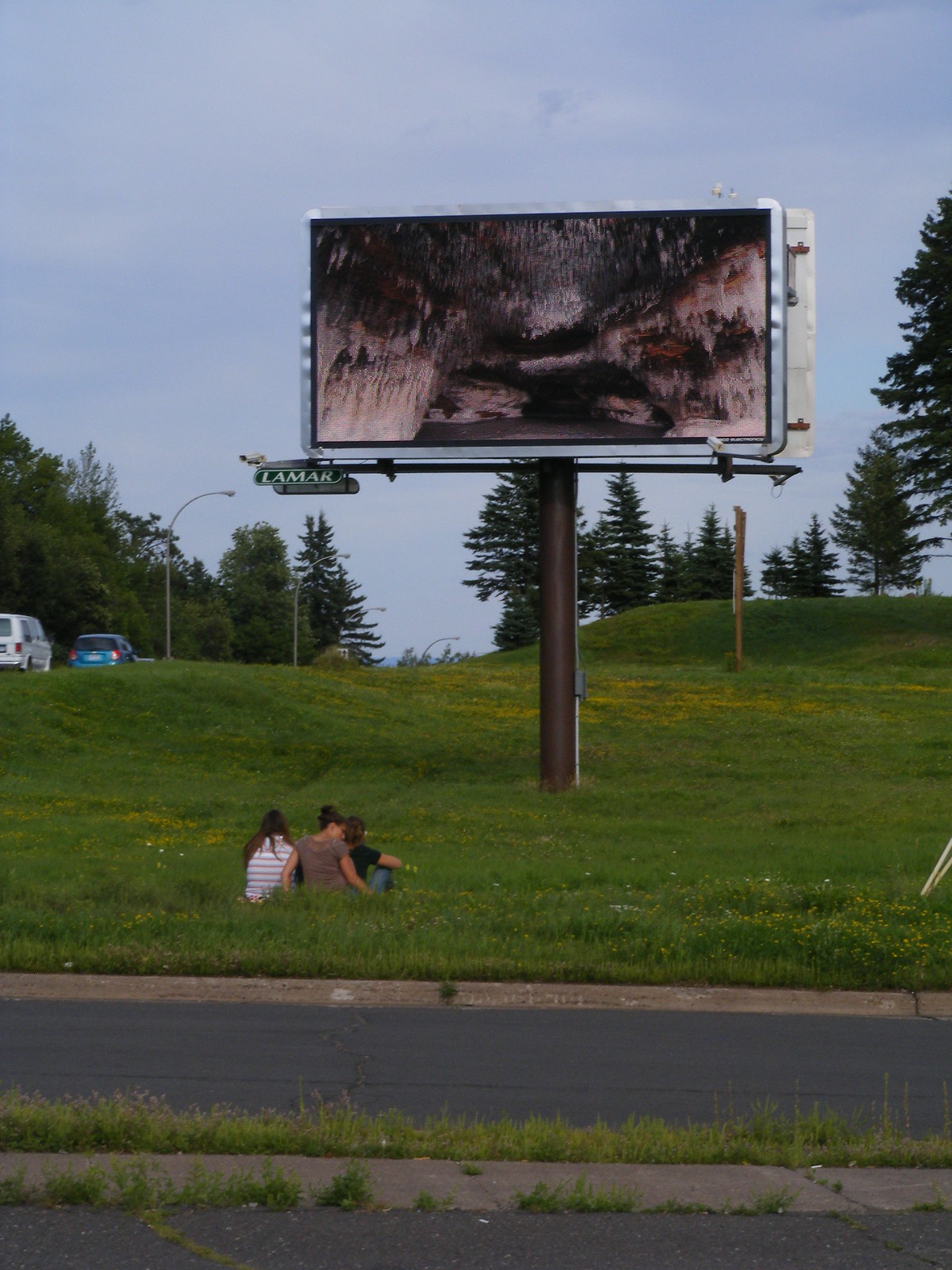The image captures a billboard mounted on a long brown pole in a grassy, hilly area near a road. The billboard displays an almost cinematic scene, depicting a dark cave with the exterior being somewhat lighter. The cave image blends hues of faded gray, black, and tan, creating an indistinct scene that feels mysterious. At the base of the billboard, a green hang sign reads "Lamar". Behind the billboard, an image seems to partially obscure the right side, indicating there might be another advertisement adjacent to it.

In the foreground, three individuals—possibly children—are sitting on the grass, gazing up at the billboard. On the left-hand side of the scene, a blue car and a white van are driving by. The road behind the children is divided by a median and features streetlights, accentuating the suburban setting. Beyond the road, a row of evergreen trees adds a touch of natural greenery to the backdrop.